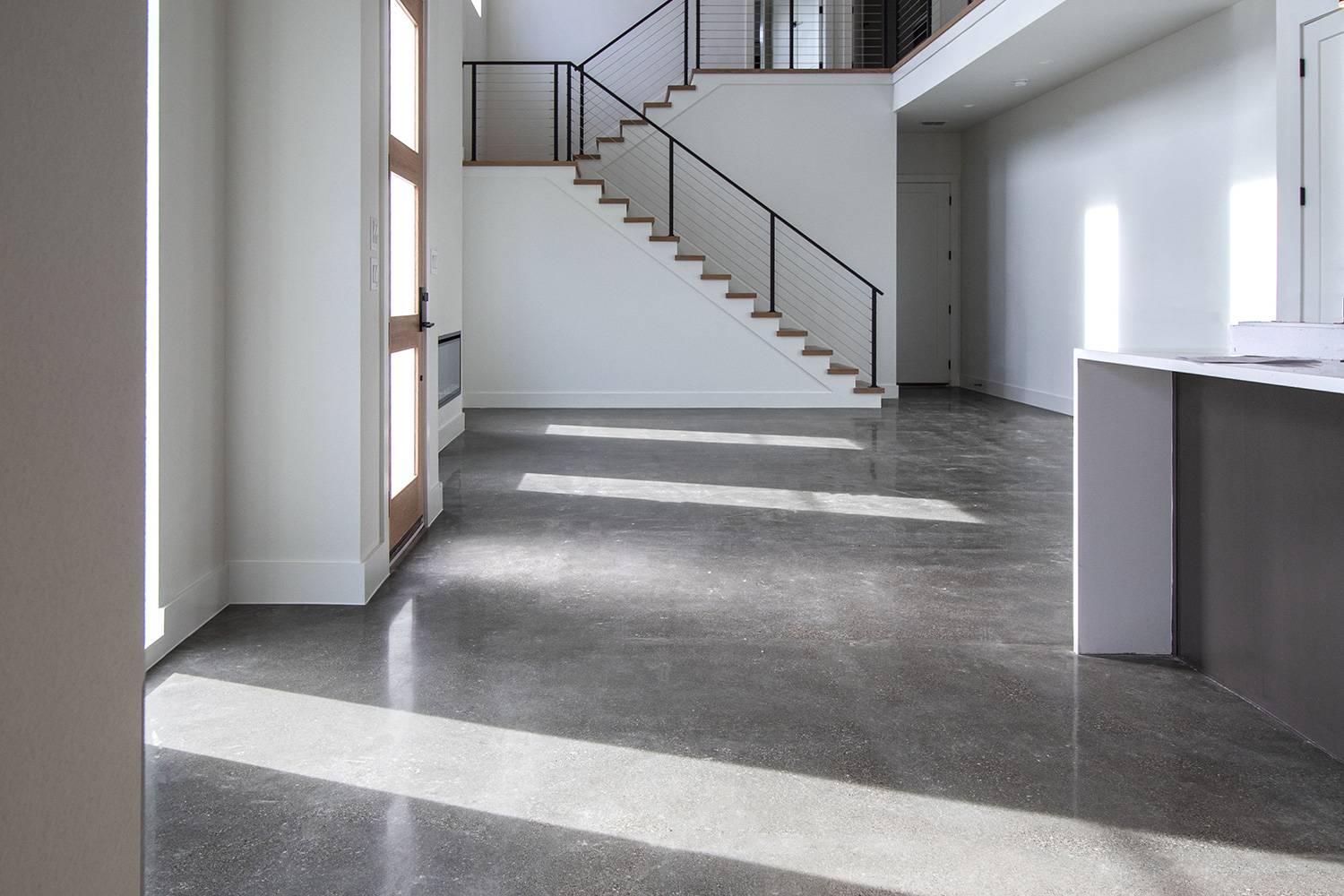This is a well-lit, professional photograph of an empty, unfurnished lobby or room, likely intended for real estate purposes. The gray floor, possibly made of polished cement or marble, extends across the room. To the left, there's a wooden door featuring three stacked glass panes. A gray and white reception desk or counter is visible in the top and bottom right-hand corners, behind which stands a blank wall. A nook in the upper section of the image leads to another door. In the background, a striking white staircase with wooden treads and a black banister features wire railings. The staircase ascends to a landing where it transitions into a second, shorter flight leading to an upper mezzanine. The entire room is illuminated by abundant natural light, casting shadows on the spotless white walls.